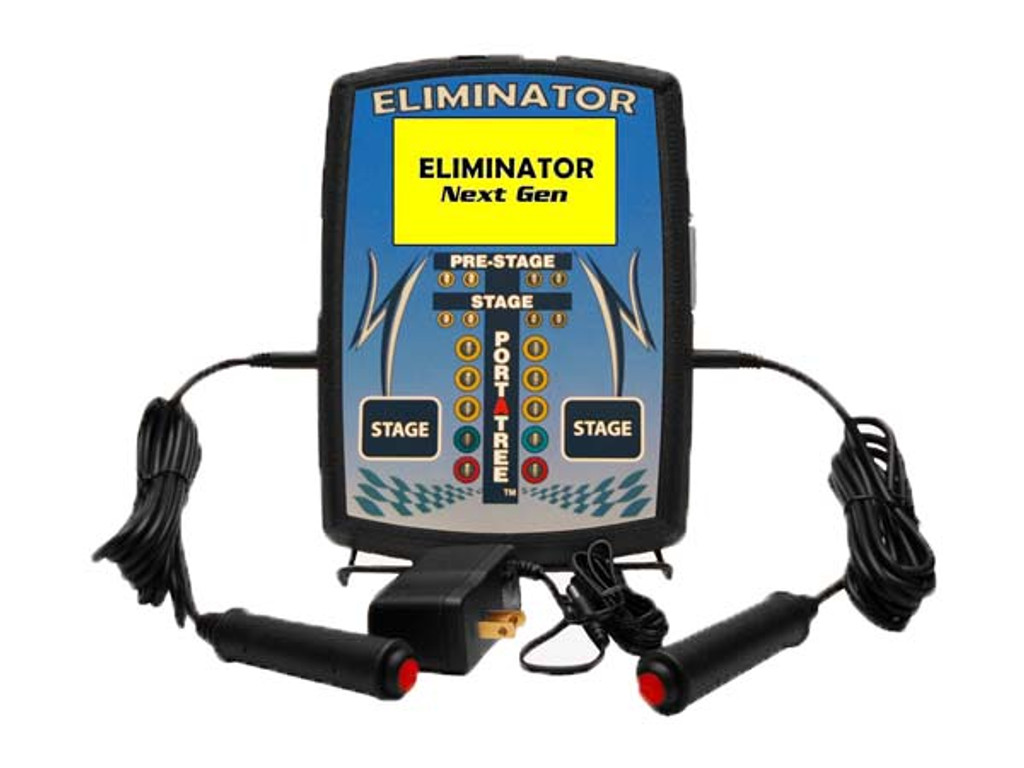In this image, a vintage electronic device sits against a plain white background. The device features a display with the word "Eliminator" in bold, capital letters at the top. Just below, in a bright yellow rectangular box, it reads "Eliminator Next Gen" in black text. Beneath this, an icon resembling a drag racing starting line tower includes labels such as "PreStage" and "Stage" in white text on a black bar. The vertical stem of the tower features the text "Porta Tree," with the "A" in "Porta" uniquely colored red. Flanking this tower are two blue boxes, each labeled "Stage" in white text. Additionally, there are several small, circular lights: two labeled "PreStage," two labeled "Stage," three yellow circles, a green circle, and a red circle, all suggesting a drag racing signal system.

From the sides of the device extend two black wires, neatly tied with twist ties, each ending in a handheld trigger with a thumb-activated red button. These seem designed to initiate some function related to the drag racing setup. A third wire emerges from the front, leading to a power adapter. The entire device, with its intricate labeling and array of signals, resembles equipment used in race track events, emphasizing both functionality and an old-school design.